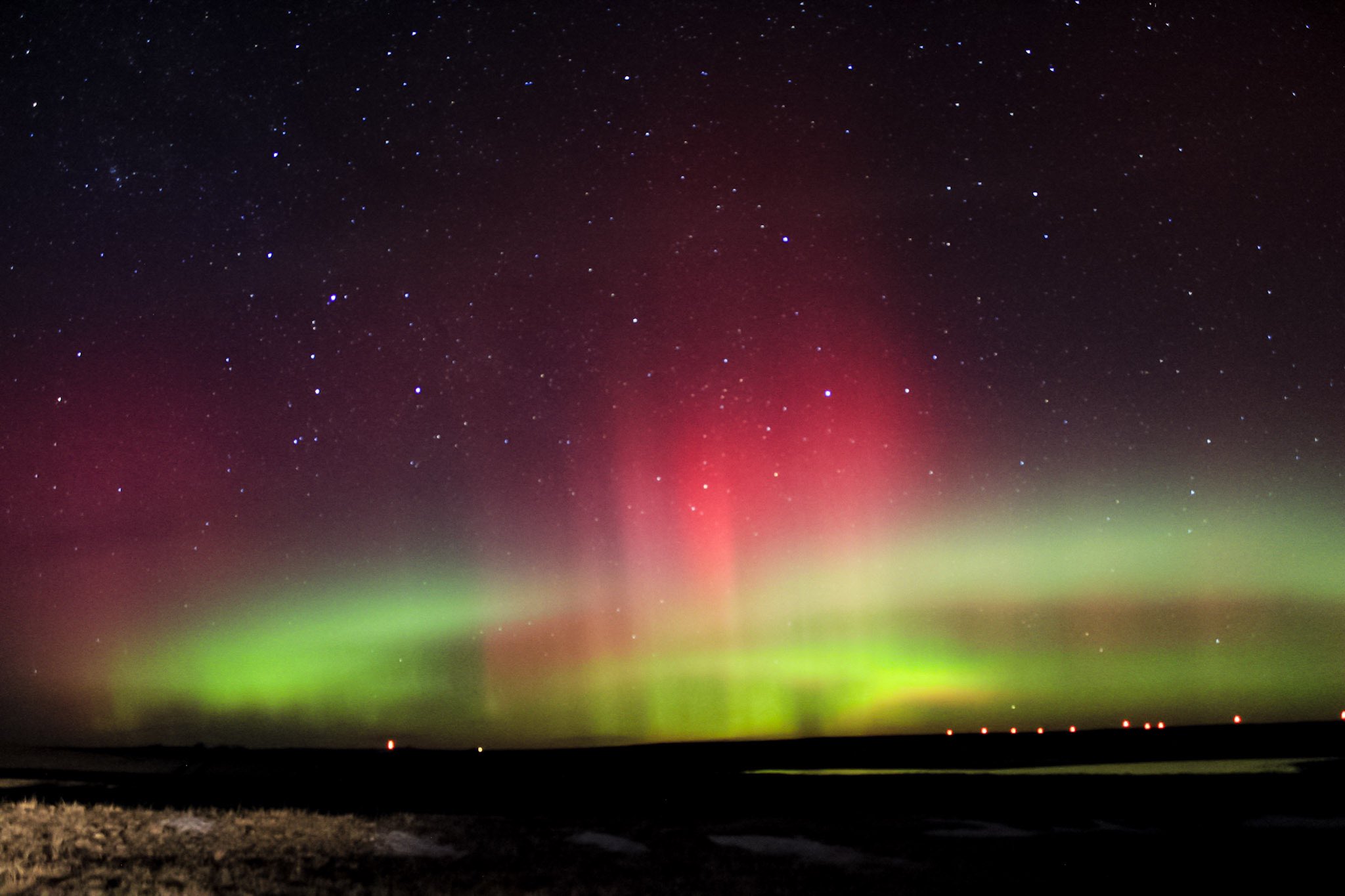The photograph captures a stunning night sky dominated by the magnificent Aurora Borealis. In the foreground, there are small rocks scattered along the shoreline, and patches of grass can be seen, possibly with a small water puddle nearby. The night sky is clear and black, sprinkled with white stars. The Aurora Borealis showcases a spectacular display of golden green and pinkish-red lights, stretching and blending upwards into the starry sky. Along the distant horizon, a few faint lights from buildings or houses are visible across a bay or body of water, adding a hint of human presence without detracting from the natural beauty. The colors of the northern lights cast subtle reflections on the ground below, enriching the photograph with a dramatic and magical ambiance.